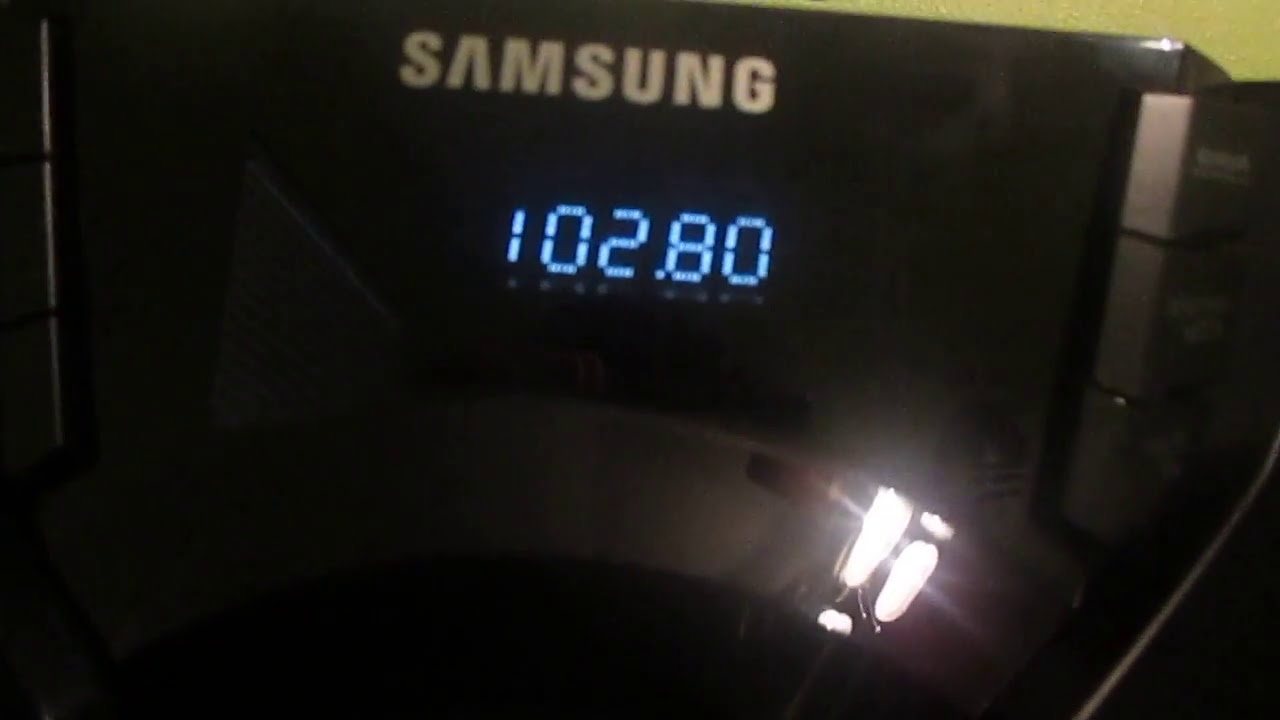The image depicts the close-up view of a black electronic device made by Samsung, characterized by its glossy plastic facade. Prominently displayed at the top center is the brand name "Samsung" in silver font against the dark background. Below the brand name is a digital readout showing the number "102.80" in blue digits, suggesting it might be an FM radio frequency. The right side of the device features a set of buttons, though their exact functions are indiscernible due to the angle and focus of the photograph. There is a pronounced reflection near the lower right quadrant, possibly caused by one or two light bulbs, casting dual bright oblong images on the device’s surface. The upper right corner of the image hints at a grayish-green background beyond the device, adding minimal context to its surroundings. The overall image is somewhat unfocused and cropped closely, making it hard to specify whether the device is a clock radio, washing machine panel, or another type of electronic product.